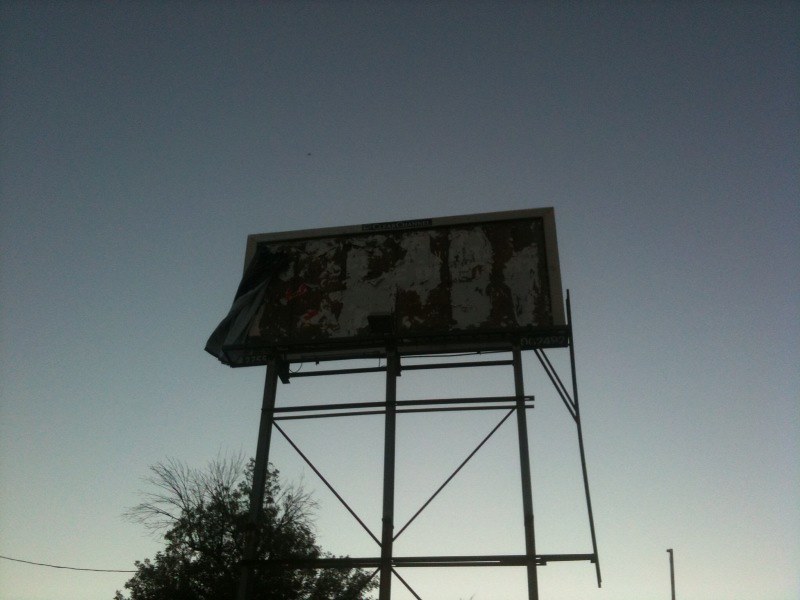The image portrays a deteriorating billboard mounted high on a metal scaffold. The billboard appears to be in a state of disrepair, with parts of its surface peeling away and some images missing. There is a visible plastic bag or some other type of material hanging off the side, suggesting that work might be underway to fix or remove it. 

A tree is growing nearby, its branches extending towards the billboard. Some branches have leaves, while others are barren. A high wire runs across from the scaffold, though its endpoint isn't visible in the image. Additionally, there is an upright pole that isn't connected to the scaffold, as well as another pole seemingly hanging off the billboard, not anchored to the ground, creating an odd, suspended effect. The entire scene hints at ongoing refurbishment efforts or preparation for dismantling.